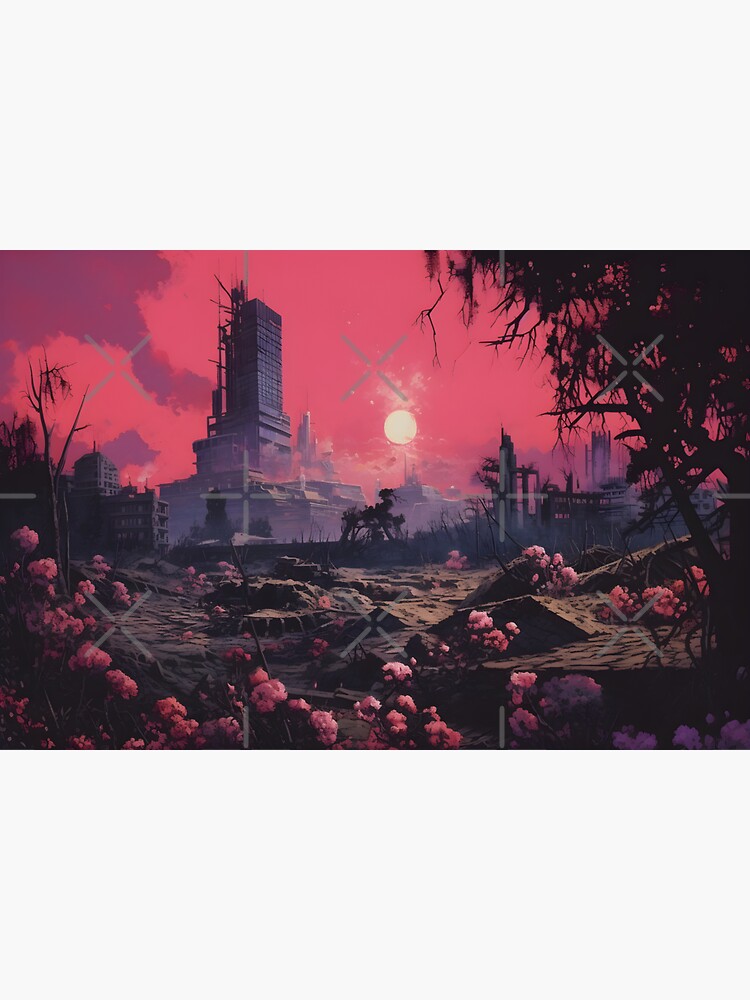The image resembles a photorealistically generated scene from either a computer-generated animated series or a video game. It portrays a city in ruins, with fallen and partially destroyed buildings, emanating an atmosphere of destruction. The sky, predominantly a vivid pink leaning towards purplish-red, features a faint, round white object – possibly a moon or sun. Emerging from an industrial plant at the top left, purple smoke swirls upwards. Scattered around the ruins are trees, bushes, and a haunting scene resembling a bombed-out landscape. In the foreground is a dirt terrain with mounds, interspersed with clusters of pretty pink flowers that contrast starkly with the devastation. A fence traverses the middle of the image, and there's an indistinct black object in front of it, further accompanied by faint gray X-shaped shadows intersecting parts of the scene. The overall hue is dominated by shades of pink and purple, imbuing the scene with an eerie, almost surreal quality.